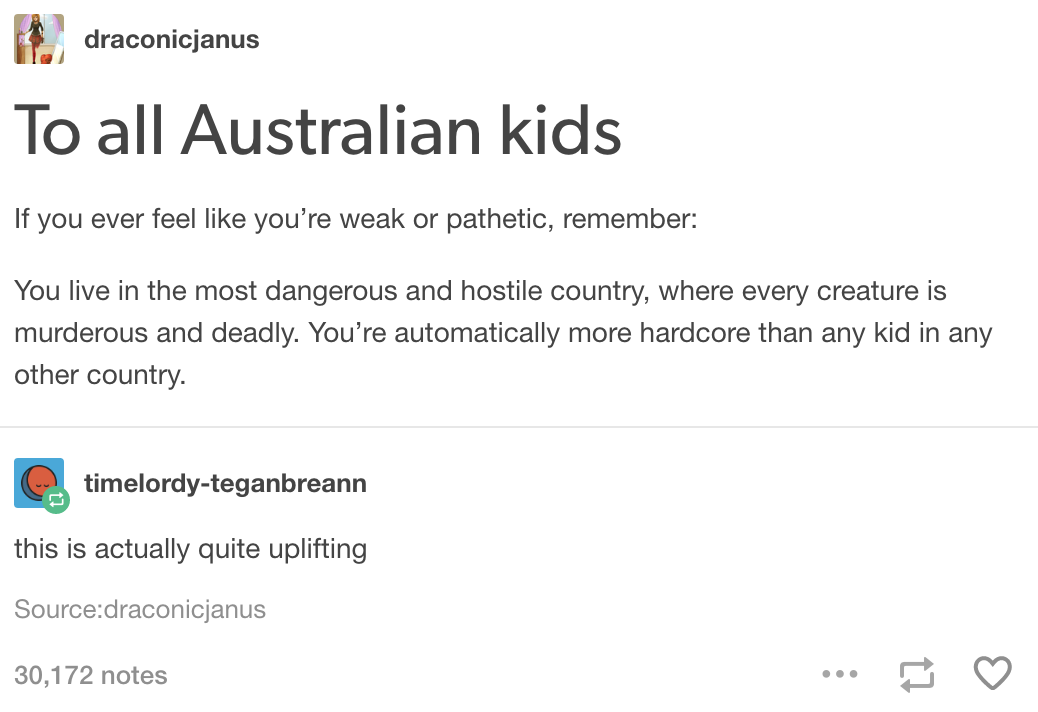**Detailed Caption:**

The image is a screenshot of a social media post. The background is predominantly white, creating a neutral canvas for the content. At the top of the image, there is a small avatar, which appears to be an anime character resembling a woman in a short skirt, although the details are vague due to the image's size. The account name, displayed prominently, reads "Draconic Janus."

The post's title, written in a large, bold font, states: "To All Australian Kids." Following the title, in smaller text, a motivational message reads: "If you ever feel like you're weak or pathetic, remember, you live in the most dangerous and hostile country, where every creature is murderous and deadly. You're automatically more hardcore than any kid in any other country."

Below this inspiring message, there is a comment from another user, whose avatar is a simple circle with two eyes. The comment, attributed to "Time Lordy Tegan Breanne," reads: "This is actually quite uplifting, Sorus Dranic Janus." 

The post has garnered significant engagement, with a count of 30,172 notes, indicating its broad reach and popularity. The overall layout suggests it is a capture of an online interaction where words of encouragement and communal support are shared.